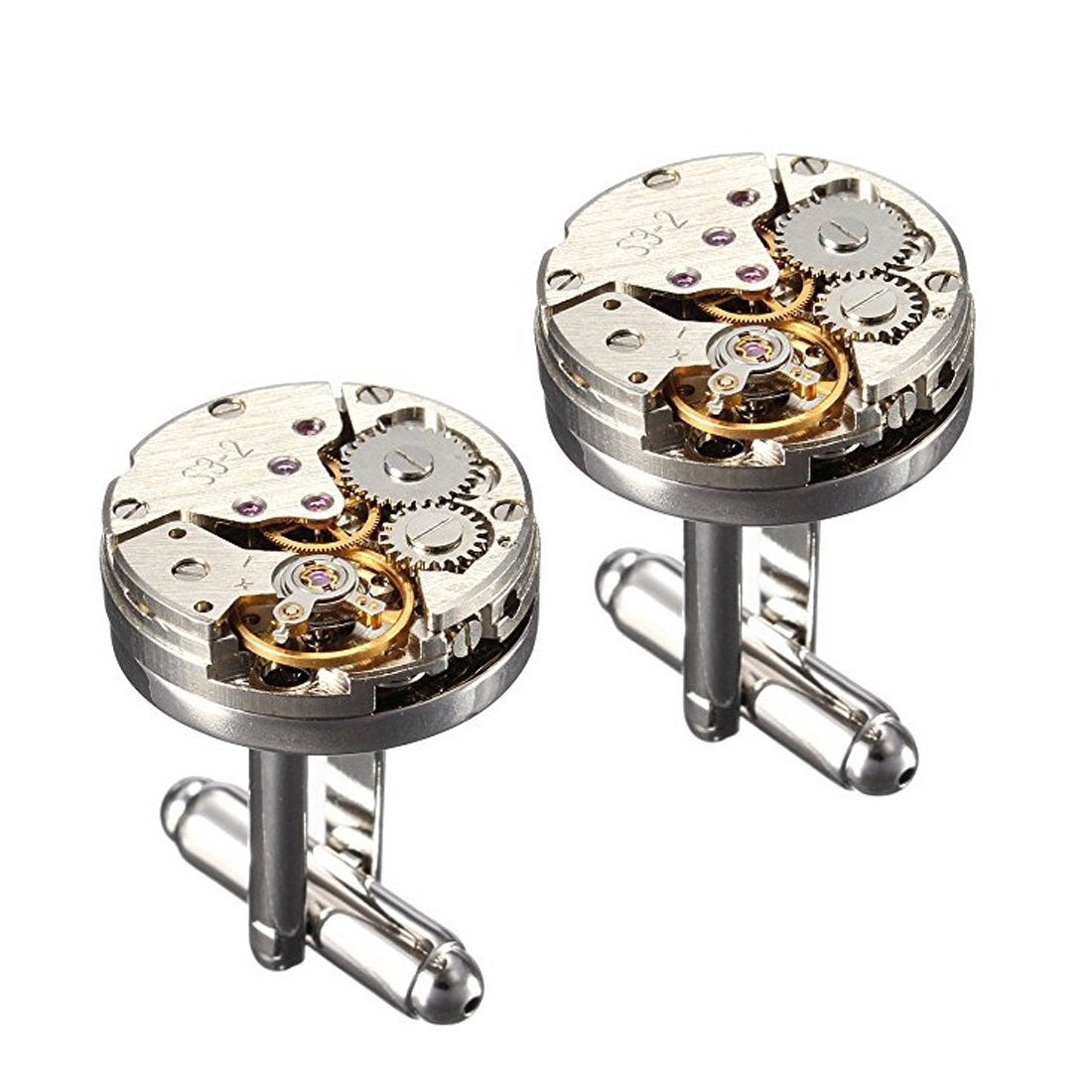This close-up photograph showcases a pair of intricately designed silver cufflinks, each featuring a miniature, mechanical aesthetic that emulates the internal mechanisms of a watch. The tops of the cufflinks display a captivating array of very small gears, screws, and other components, meticulously resembling the intricate details you would see if you opened the back of a watch. The mechanism includes both silver and gold gears—specifically, two silver gears and two gold ones—adding a touch of luxury to the overall design. An additional detail includes a small, yet distinguishable, pink or purple element embedded within the mechanism. The cufflinks also feature precise engravings: the number 'S3-2' and tiny plus and minus symbols, lending a further air of technical sophistication to these stylish accessories.